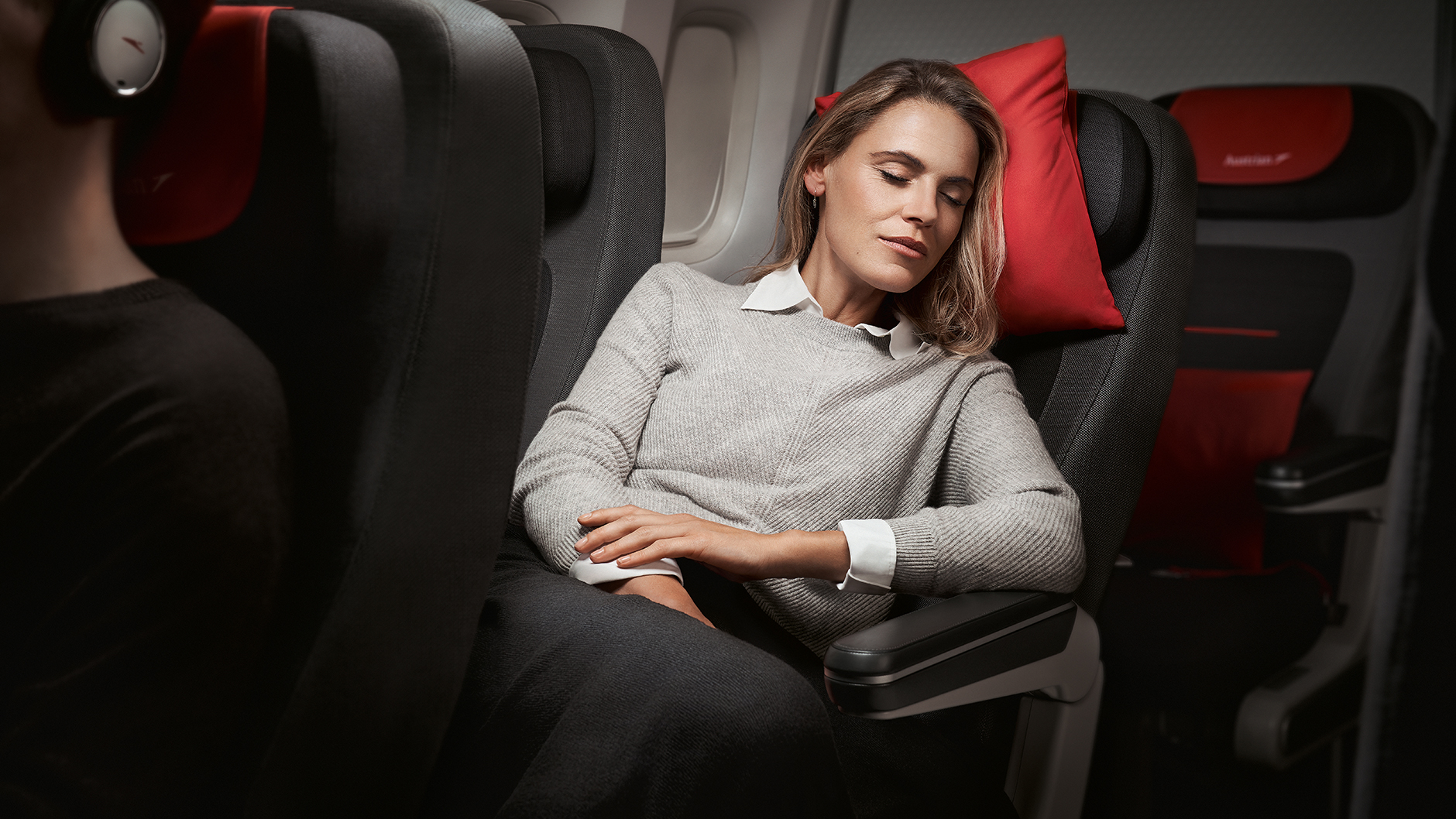A blonde woman is asleep on an airplane, resting her head on a small red pillow against the headrest of her black seat. Her body is facing the aisle, with her head tilted slightly to the right. She's wearing a three-quarter length light gray sweater over a white shirt, with the collar and sleeves peeking out, and black pants. Her right arm rests on the armrest, while her left hand is tucked between her crossed legs. The airplane seats have black and red upholstery—black overall with red headrests and backrest bottoms, which are more visible on the empty seat behind her. Above the sleeping woman, another passenger’s shoulder and dark shirt, along with headphones, can be seen. The small, oval-shaped airplane windows, with one partially covered by a curtain, confirm the setting is an airplane. The soft glow of a night light illuminates the woman, while the seats around her appear unoccupied, indicating a quiet, undisturbed flight.